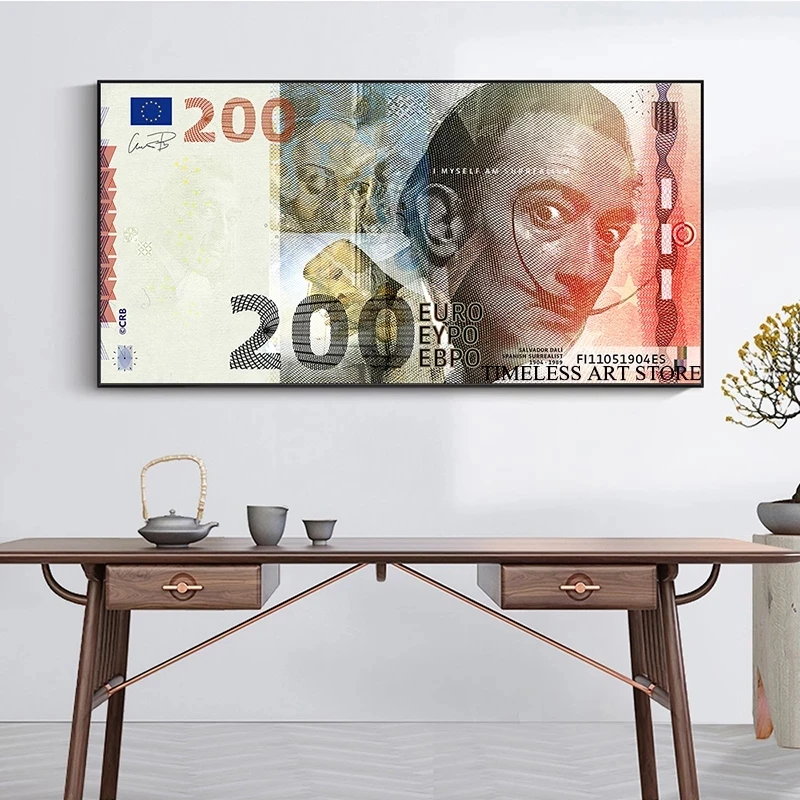The image depicts a uniquely designed wooden table with a bronze finish, featuring two built-in shelves at the bottom. Atop the table is a small tea set, comprising a grey pot and matching grey cups. The table is positioned in a minimalist room with light grey, angular patterned flooring and a white-painted wall. Dominating the wall behind the table is a large, blown-up reproduction of a 200 euro note. This note prominently features Salvador Dali, recognizable by his trademark giant waxed mustache and wide-eyed, surprised expression. The note includes a partially readable phrase, "I myself am," and in the bottom right corner, it reads, "timeless art store." The picture is enclosed in a thin black border. Adjacent to the table, on the right side of the image, is a small bonsai tree with yellow leaves. The overall setting resembles an elegantly styled living room or foyer, showcasing a cohesive blend of art and interior design.